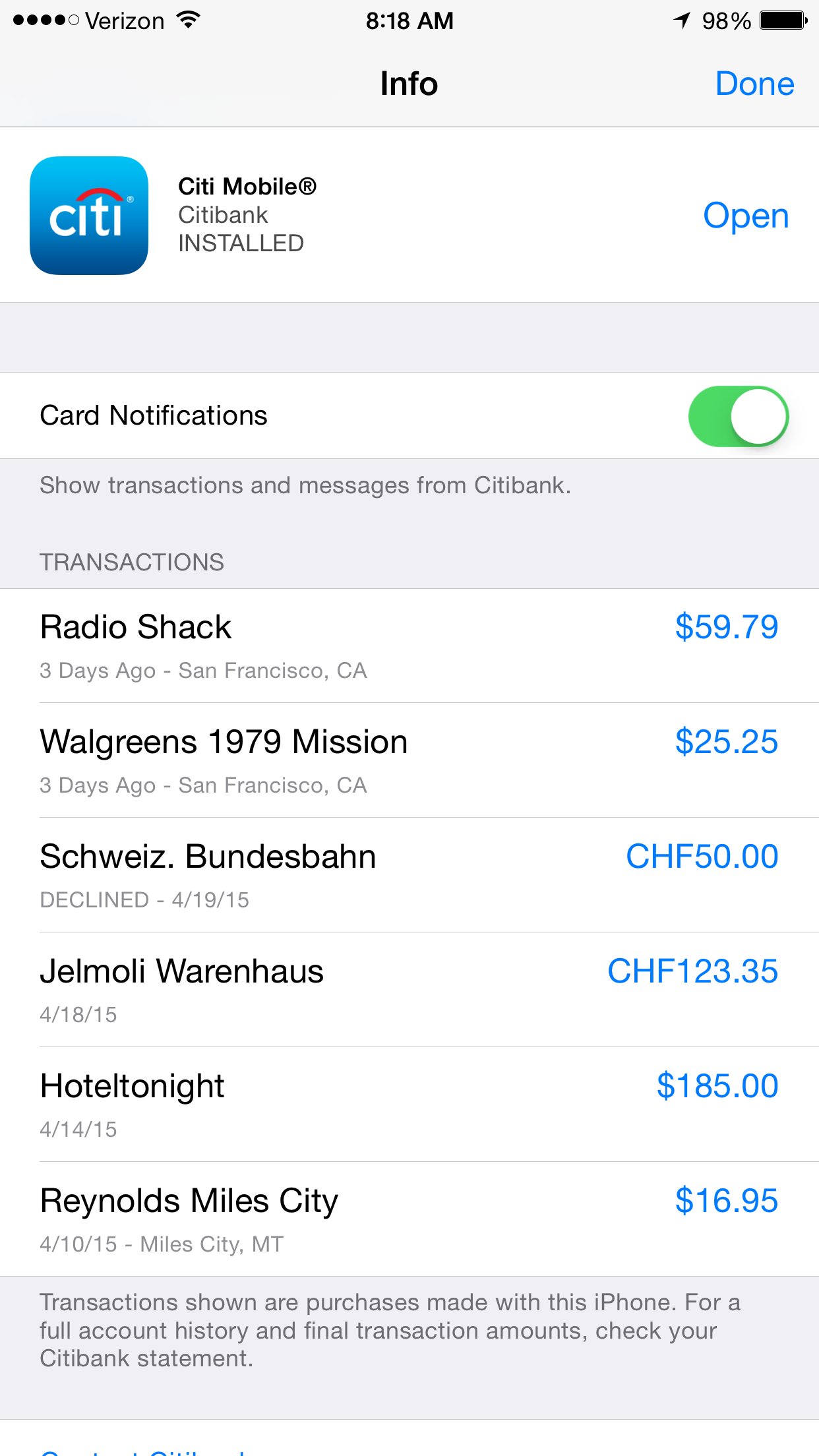The screenshot displays a smartphone interface set against a white background. In the upper left corner, the screen indicates a strong signal with four out of five circles for reception, and the Verizon Wi-Fi icon is illuminated. It is 8:18 a.m., and the battery is at 98%. 

In the center, the word "Info" is visible, with "Done" in blue text positioned to the right. Below this, the "City Mobile" app icon is displayed, and to the right, it reads "City Mobile Citibank installed." 

Further down, there is a section for card notifications with a toggle switch to the right, which is turned on. This section shows transactions and messages from Citibank, with a list of transactions displayed as follows:
- Radio Shack: $59.79
- Walgreens: $19.79
- Mission San Francisco California: $25.25
- Schweiss Bunzbahn: CHF $50 (declined)
- $4.19, 15 Jamali Warenhaus: CHF $123.35